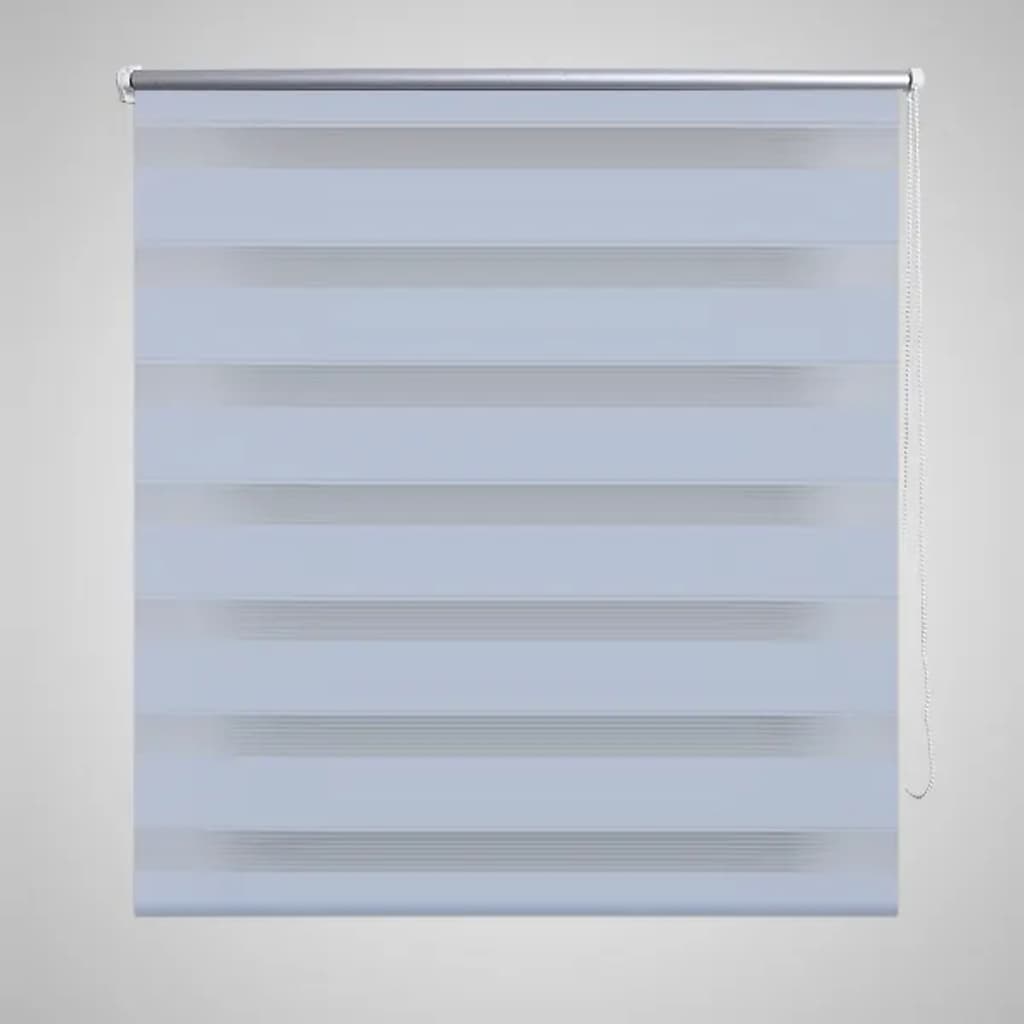The image centers on a prominent, highly detailed window shade that occupies most of the frame, with an eggshell or light gray background. The shade itself is a light, powder blue with subtle gray undertones, and it features seven vertical stripes running down its length. Suspended from a silver metallic pole at the top, which is secured to the wall with white clips on either side, the shade is intricately designed. To the right, a metal pull cord hangs, reminiscent of those found on older pull-cord light bulbs. Though depicted with lifelike texture and color, there is a distinct impression that the image might be a digital or computer-generated render, particularly due to its highly polished and somewhat surreal appearance.